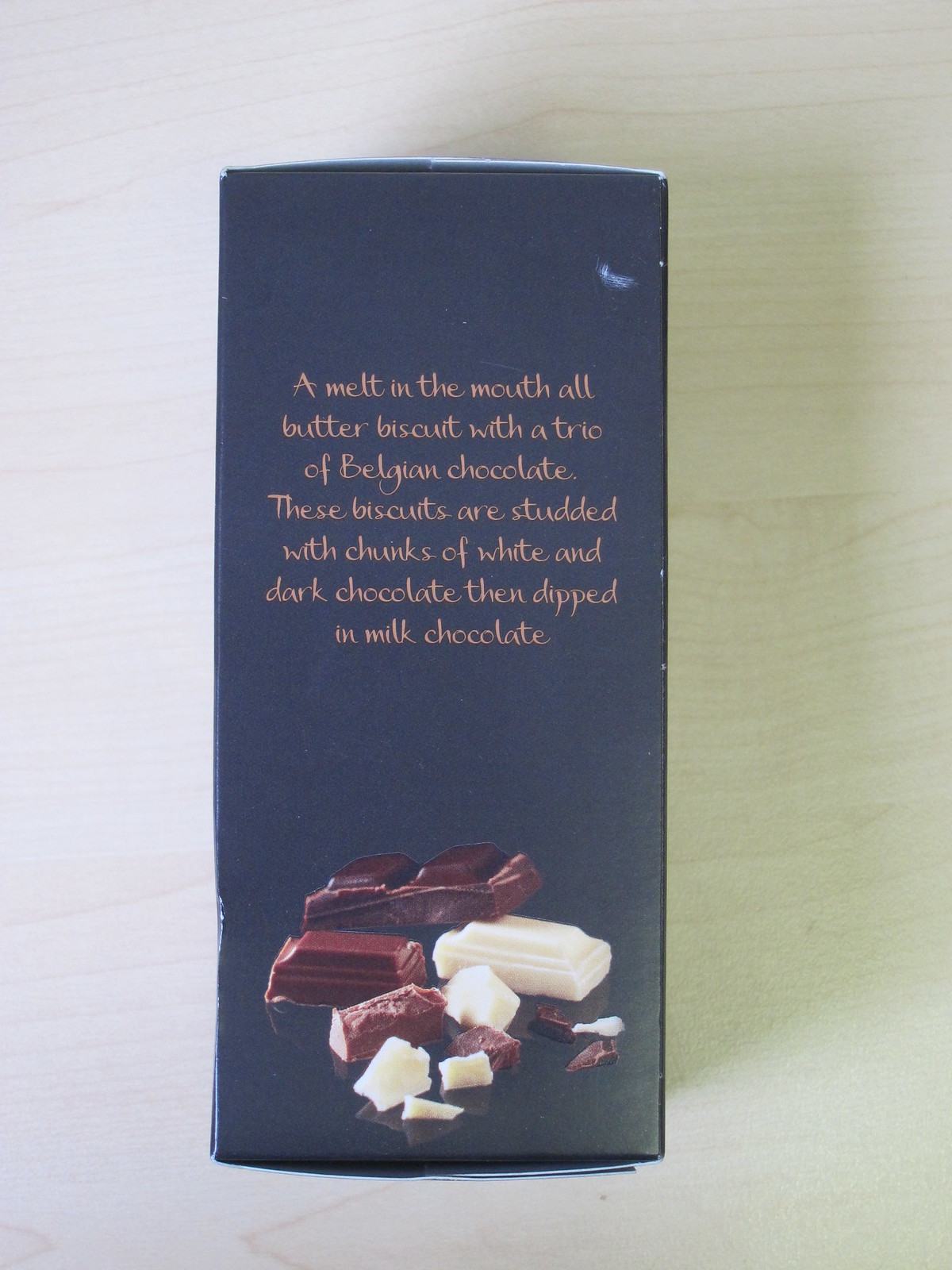The image features a rectangular, black box resting on a tan, wooden table. The box prominently showcases gold or light brown writing that reads, "A melt-in-the-mouth all-butter biscuit with a trio of Belgian chocolate." These indulgent biscuits are described as being studded with chunks of both white and dark chocolate, then dipped in milk chocolate. Toward the lower section of the box, there are images of pieces of dark and white chocolate. The composition is viewed from above, with the shadow of the box cast to the upper right. The table’s wood grain and the color palette—consisting of blacks, golds, browns, whites, and tans—enhance the luxurious presentation of the product. There are no visible people or additional text in the image, highlighting the product as the central focus.